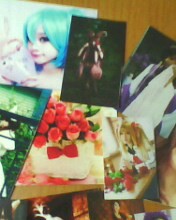In this somewhat blurry mosaic, various images are juxtaposed, creating a collage of intriguing details. In the upper left corner, a young child with alabaster skin, striking black eyes, and striking teal hair is prominently featured. Just to the right of the child, amidst a background of lush vegetation, is a photograph featuring what appears to be a pink flamingo, though on closer inspection, it may actually be a person riding a pink bicycle.

Central to the composition is a cake adorned with a meticulously tied red bowtie and garnished with delicate pink and purple flowers atop its white frosting. The cake is set upon a light wood-colored table, enhancing its visual appeal.

To the left of the cake, a series of photographs lean against a brown wall. One photograph, predominantly dark with hints of orange and purple at the bottom, is indistinct. Directly below, another photograph portrays a blonde-haired woman staring intently forward.

In the extreme left corner of the image, another picture pierces the frame, dominated by a light green hue accented by descending black lines. This detailed collection of images melds together, telling a vibrant, if somewhat obscured, story.